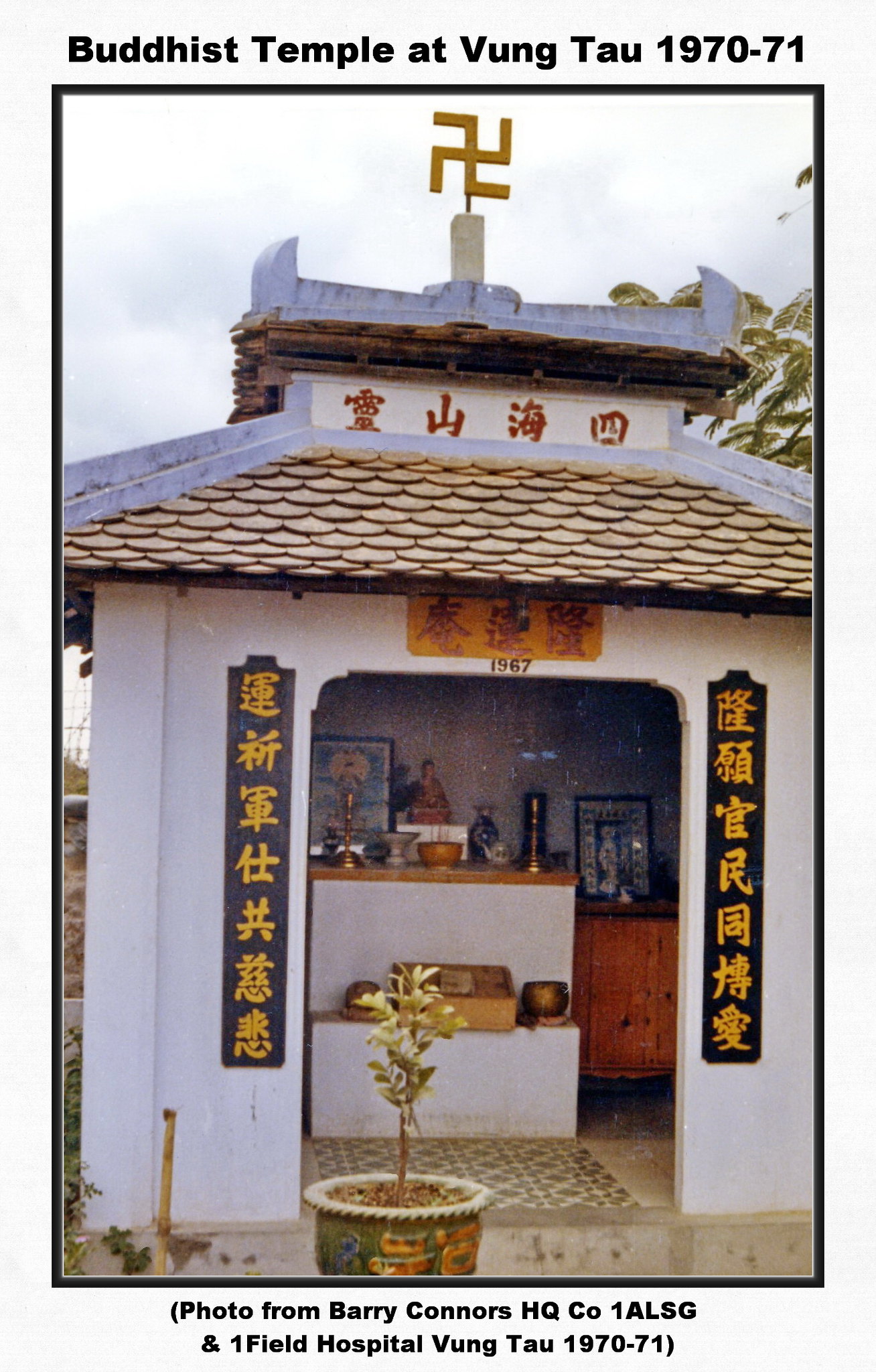This outdoor photograph, formatted like a postcard with a white border and a thin black pinstripe, is of a Buddhist temple at Vung Tau in 1970-71. The white border contains a caption at the top stating, "Buddhist Temple at Vung Tau, 1970-71," and at the bottom, in parentheses, "photo from Barry Connors, HQCO 1ALSG and Field Hospital, Vung Tau, 1970-71." The temple is a small, single-room white building with wooden shingles that resemble light brown scales. The roof has slanted sides, and above it is a protruding top portion featuring a reversed Buddhist swastika in gold. 

The front entrance is a large opening with beveled sides, dated 1967 above the doorway. Flanking the entrance are black vertical banners with gold Chinese lettering. In front of the entrance sits a small tree in a green pot, and inside the building, various decorations, figurines, and photographs are arranged on white tables. The image, taken on an overcast day, captures the intricate details and serene ambiance of the temple.